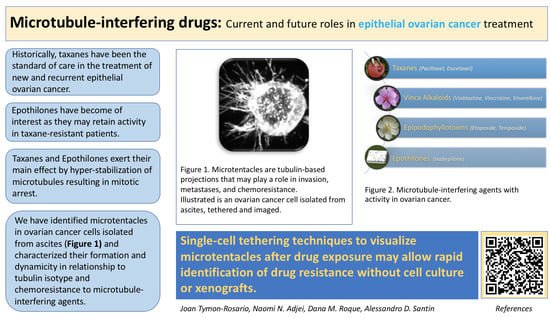The image is a detailed diagram from a medical webpage, focusing on “Microtubule-Interfering Drugs: Current and Future Roles in Epithelial Ovarian Cancer Treatment,” as indicated by the yellow title box at the top. The left side of the image features four blue bubbles with rounded corners, providing historical and current insights into the use of taxanes and epothilones in treating epithelial ovarian cancer. Specifically, the text explains the traditional reliance on taxanes, the potential of epothilones in taxane-resistant cases, and the mechanism by which these drugs work—hyperstabilizing microtubules to induce mitotic arrest. Additionally, the bubbles discuss the identification of microtubules in ovarian cancer cells isolated from ascites, their formation dynamics, and resistance to microtubule-interfering agents.

The center of the image showcases Figure 1, a black-and-white depiction of an ovarian cancer cell with tubulin-based microtentacles. This figure emphasizes the role of microtentacles in invasion, metastasis, and chemoresistance. Directly below this figure, a blue text box highlights the significance of single-cell tethering techniques in visualizing microtentacles post-drug exposure for the rapid identification of drug resistance without the need for cell culture or xenografts.

To the right of Figure 1, there is an illustration labeled as Figure 2, depicting various microtubule-interfering agents categorized into taxanes, vinca alkaloids, epothilones, and photolines, though the text here is harder to read. At the bottom right corner, a QR code provides references, and the image credits research contributors Joan Tyman-Rosario, Naomi N. Adjaye, Dana M. Roque, and Alessandro D. Santin.